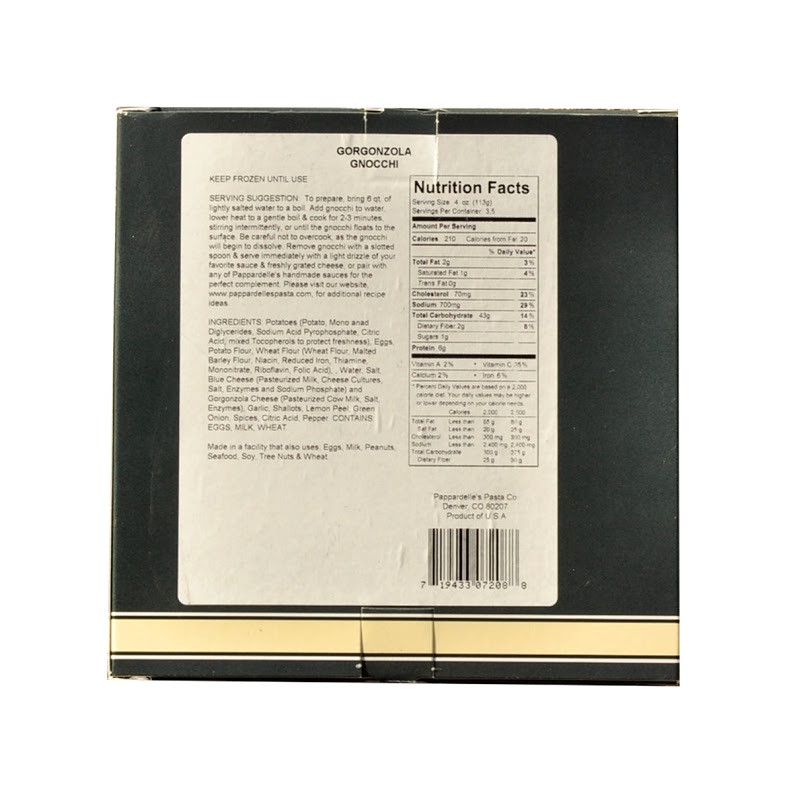This detailed image features the back label of a food item, specifically Gorgonzola Gnocchi. The label, black and white in design, sits against a larger black package with a distinct beige stripe running horizontally at the bottom, bordered by two thin black lines. The label is divided into two primary columns. 

The left column provides storage instructions, advising to keep the item frozen until use, along with serving suggestions for preparation. Below this section, there is a list of ingredients included in the product. 

On the right column, detailed nutrition facts are presented, listing information such as the amount per serving, which is a 4-ounce portion containing approximately 275 calories, 7 grams of fat, 75 grams of carbohydrates, and 4 grams of protein. It also notes additional nutritional information such as sodium, cholesterol, and total daily value percentages. 

At the very bottom right corner of this label is a barcode. While some finer details remain unreadable, the label indicates that the product is made in the USA, specifically in Denver, Colorado, although the exact company name is not clear. This thorough description on the packaging provides consumers with essential information about the Gorgonzola Gnocchi, covering storage, preparation, ingredients, and nutritional content.